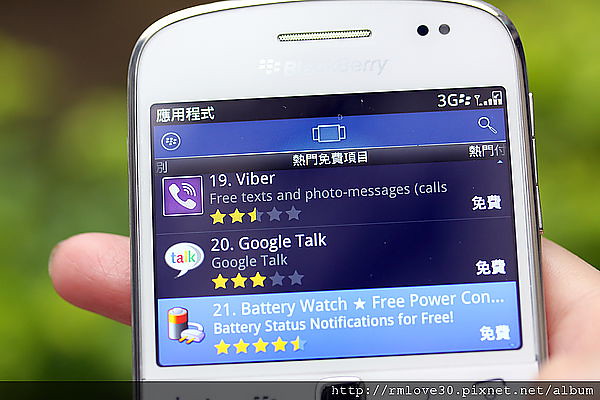A close-up photo depicts a hand holding a BlackBerry phone against a backdrop of blurry green foliage, suggesting an outdoor setting. The focus is on the phone, which is white with "BlackBerry" written in silver at the top. The upper-left corner displays some Asian characters, while the top-right corner shows "3G" and signal bars indicating internet connectivity. Additionally, there's a battery icon next to these indicators. Three applications are listed on the screen: "19 Viber" with a purple icon and 2.5 stars, "20 Google Talk" with 3 stars, and "21 Battery Watch" with 4.5 stars. The phone's screen and text are mostly in English, although some lines of Asian script are evident. The user's hand, partly visible, holds the device securely.